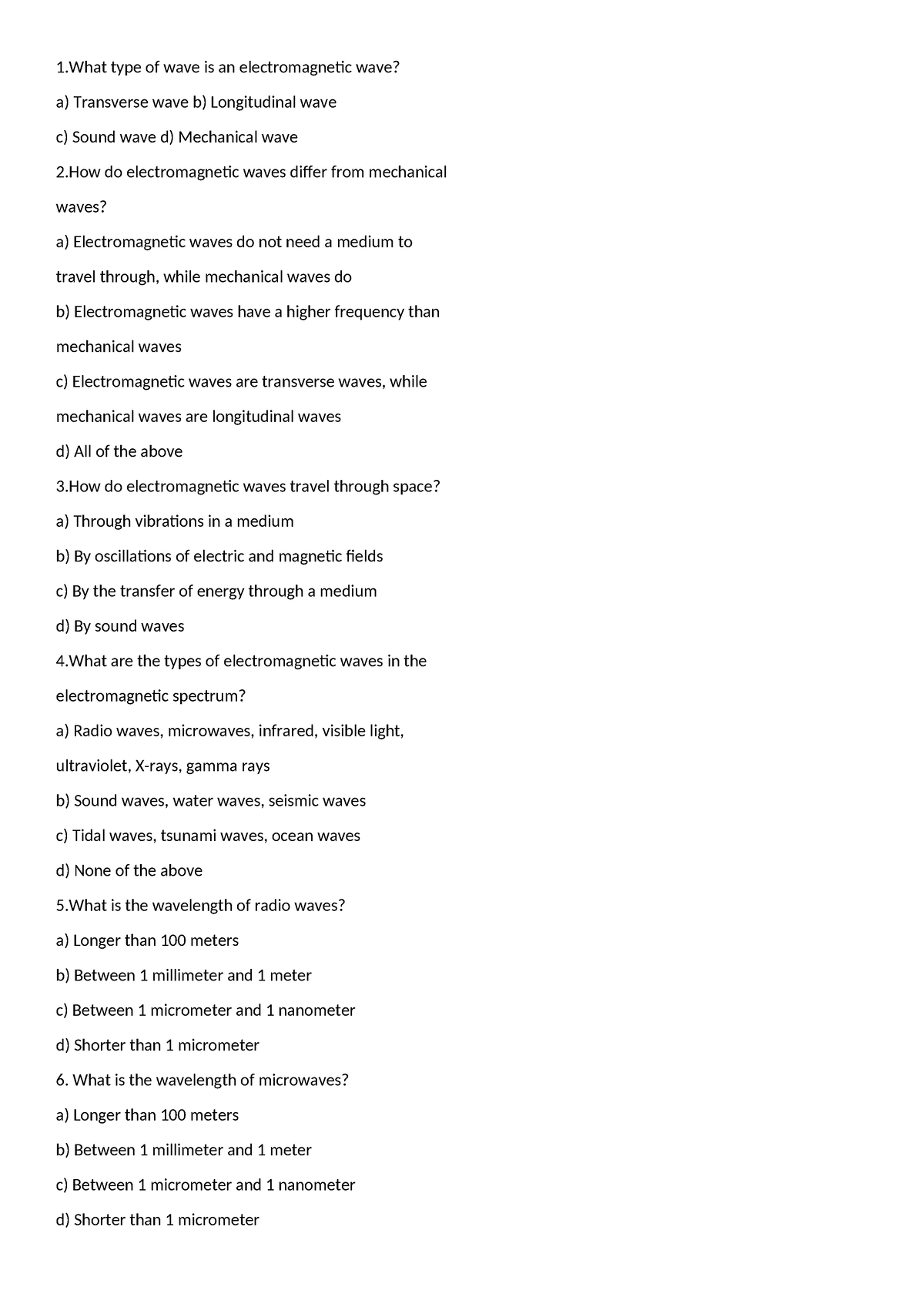**Detailed Descriptive Caption**:

This image illustrates the various types of waves, including electromagnetic waves, transverse waves, longitudinal waves, sound waves, and mechanical waves. It delves into the fundamental differences between electromagnetic and mechanical waves. While electromagnetic waves, which are transverse waves, do not require a medium for travel and have a higher frequency, mechanical waves (such as sound waves, which are longitudinal) do need a medium to propagate. Moreover, electromagnetic waves travel through space via oscillations of electric and magnetic fields, independent of any material medium.

The image also highlights the types of electromagnetic waves in the electromagnetic spectrum, such as radio waves, microwaves, infrared, visible light, ultraviolet, X-rays, and gamma rays, and contrasts these with various non-electromagnetic waves like sound waves and ocean waves.

Additionally, the image provides information about the wavelengths of different electromagnetic waves. For example, radio waves have wavelengths longer than 100 meters, whereas microwaves have wavelengths ranging between 1 millimeter and 1 meter.

Transcribed by Otter.ai